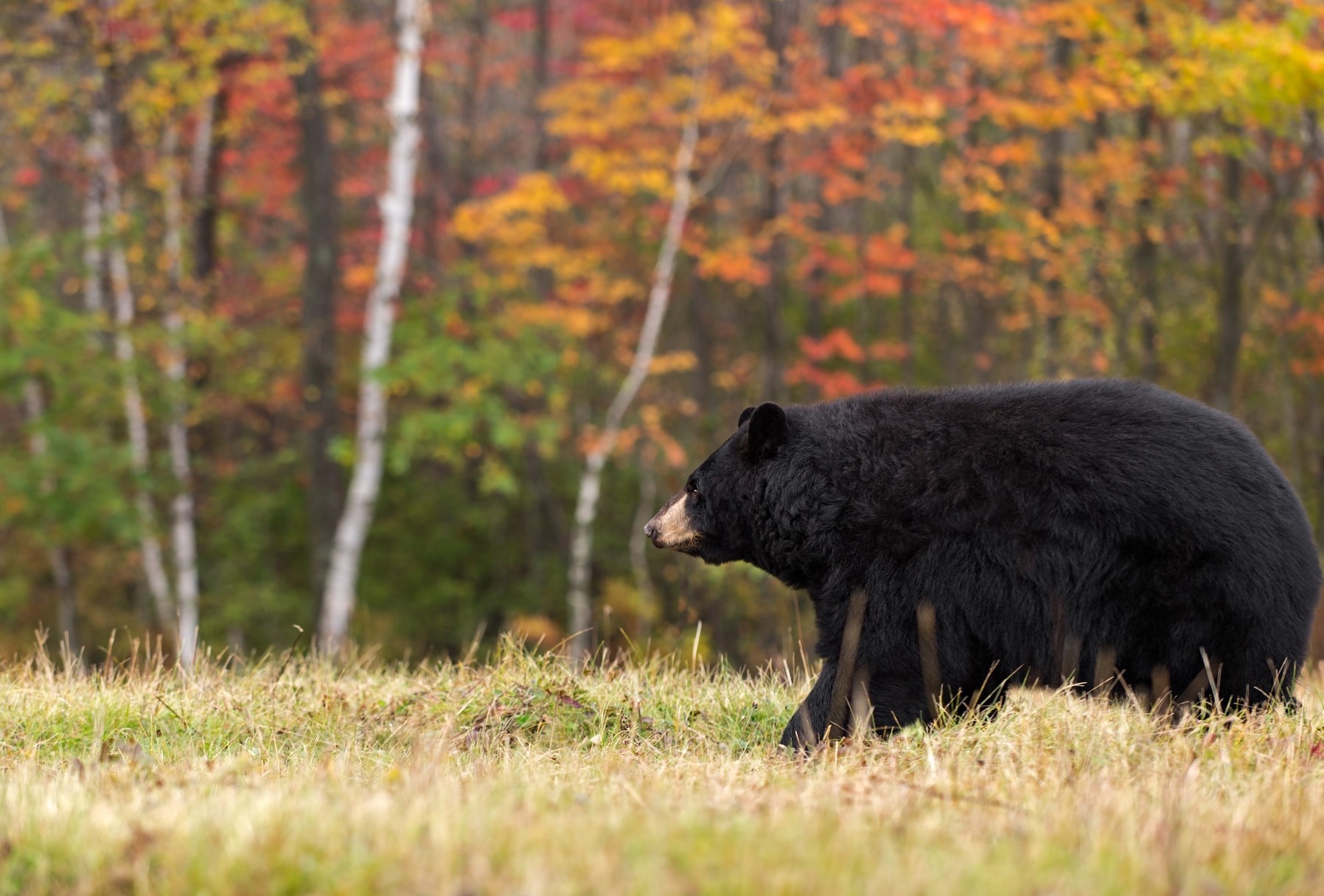In this detailed nature photograph captured during early autumn, a black bear is prominently featured, standing and walking through a tall, grassy field that transitions in color from green to brown, indicative of the season. Positioned on the right side of the image, the bear's dark black fur contrasts with the lighter brown hues on its face. The background, although blurred with a bokeh effect, reveals a dense forest adorned with trees bearing vibrant yellow, red, and green leaves, suggesting peak fall foliage. Some of the trees have distinctive white bark, contributing to the picturesque autumnal scene.